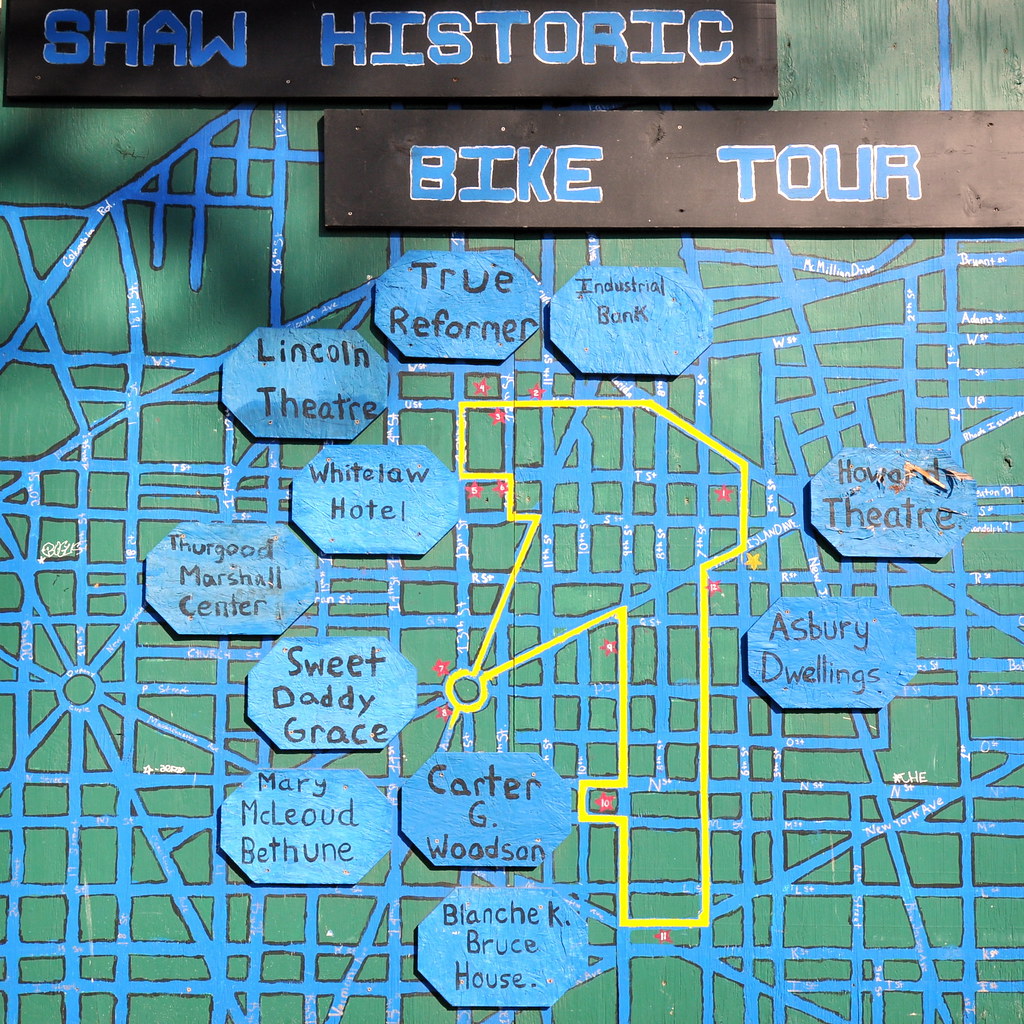This image depicts a detailed, handmade map mounted on a green-painted wooden board, with sunlight casting shadows that suggest the presence of nearby leaves. At the top of the map, a black rectangle displays the title "Shaw Historic Bike Tour" in bold blue lettering. The map itself shows a network of crisscrossing blue lines representing streets, some of which include illegible white street names. A yellow highlighted path winds through the center of the map, indicating a specific route. Key points along this route are marked with red stars, and above each star is a blue octagonal shape containing the name of a landmark. Notable destinations indicated on the map include Industrial Bank, Lincoln Theatre, Asbury Dwellings, True Reformer, Howard Theatre, Carter G. Woodson, Blanche K. Bruce House, Mary McLeod Bethune, Sweet Daddy Grace, Thurgood Marshall Center, Whitelaw Hotel, and Lincoln Theatre. Shadows at the top right reveal the texture of the wooden board beneath the green paint, adding to the rustic charm of the display.